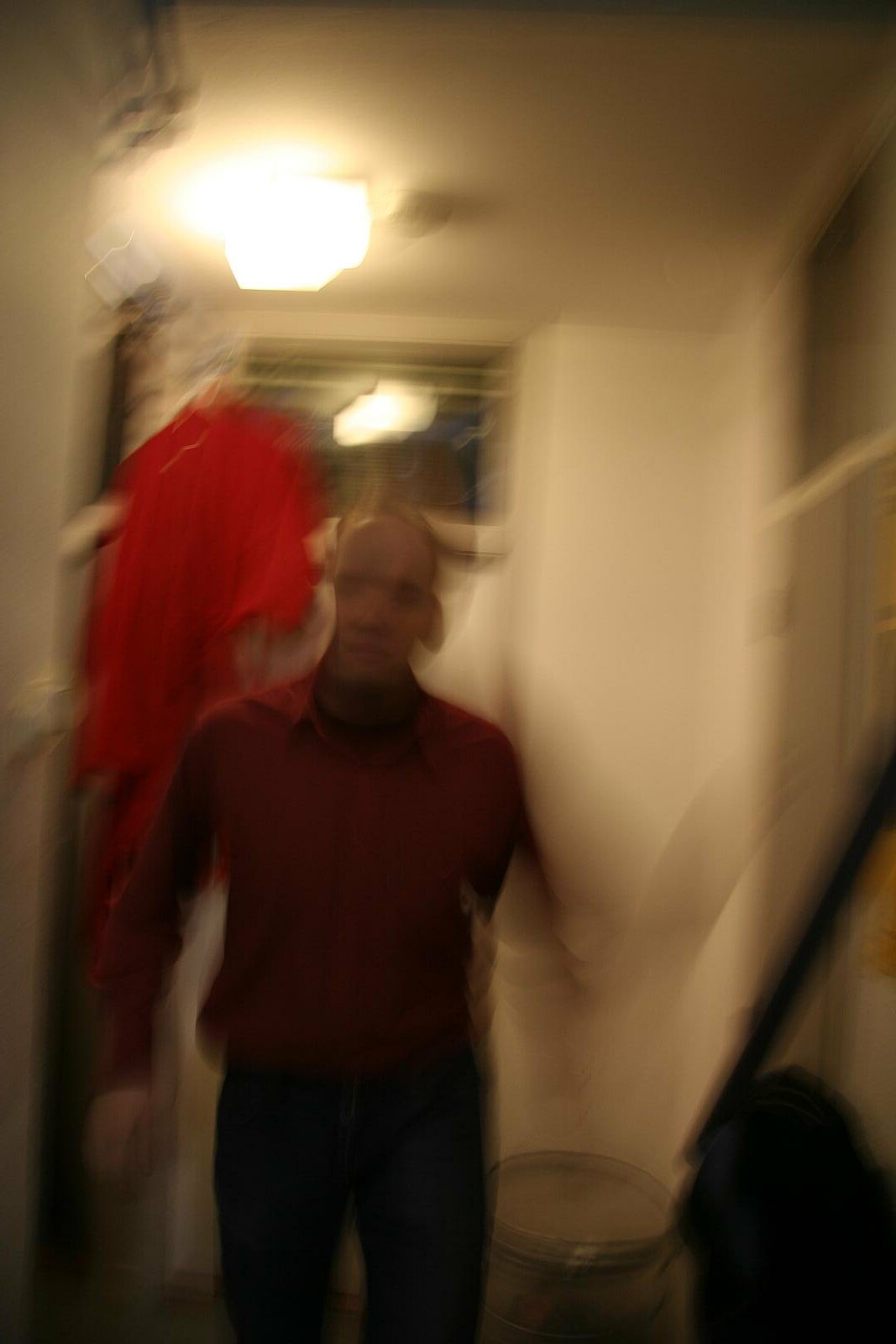The image, albeit blurry, captures a man standing in the brightly lit entry hall of a home. The overhead light casts a clear illumination in the room, highlighting the white walls and the wooden handrail of a staircase to his left. The front door behind him features a window that reflects the light, adding to the room’s brightness. The man appears to have just entered, possibly from outside. He is wearing dark pants and a wine-colored shirt with a collar, layered over what seems to be a turtleneck. His bald or balding head is noticeable, and while one of his arms rests at his side, the other is moving, creating a blur as if he’s in the midst of gesturing. Near the top of the door frame behind him, a red item—likely a shirt or a coat—is hanging prominently, adding a splash of color to the scene.